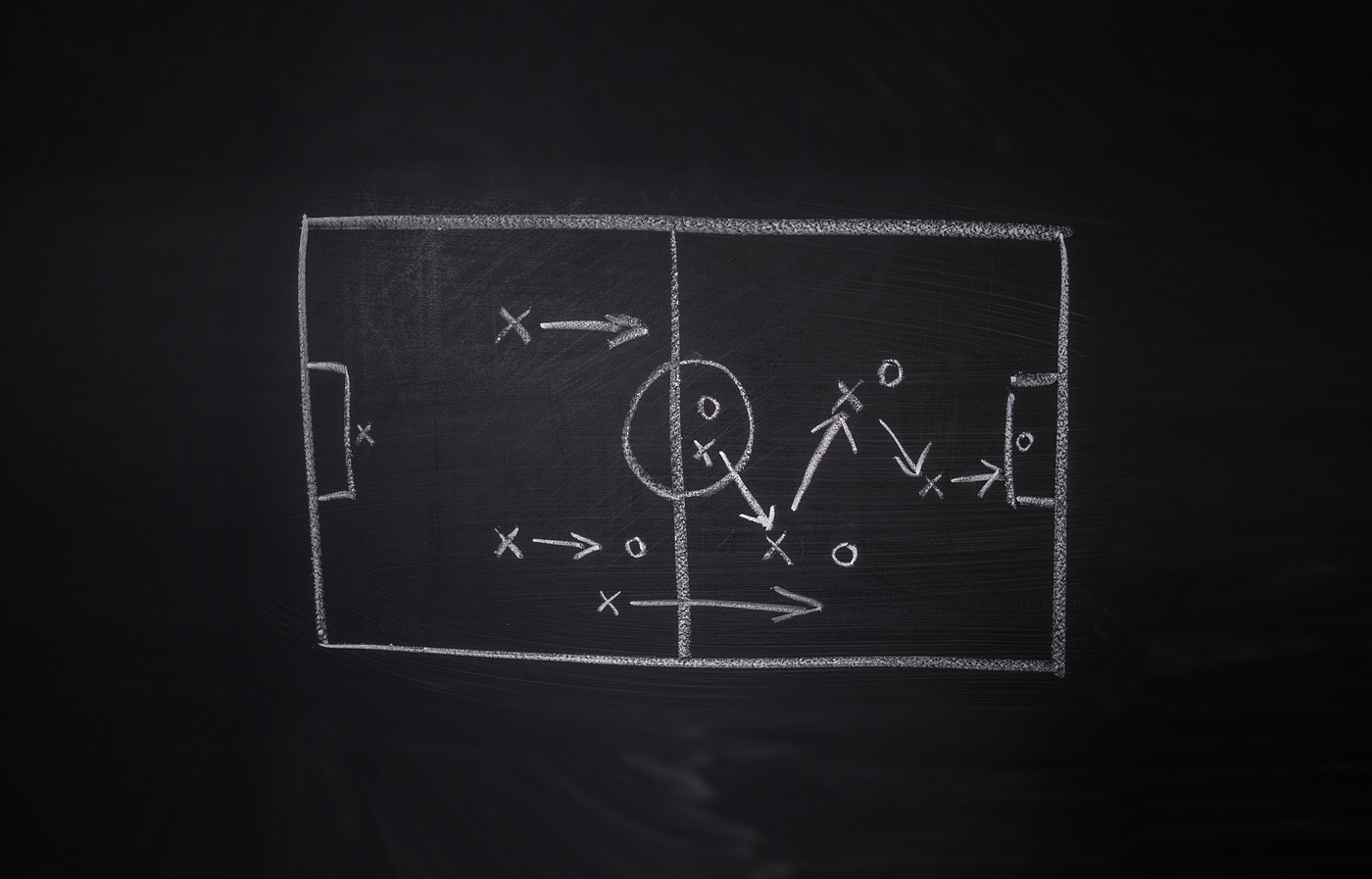The image depicts a detailed white ink drawing on a black or grayish-blue background, resembling a chalkboard used by a soccer coach. The drawing is a rectangular representation of a soccer field, complete with markings for the center line and goals at either end. Xs and Os symbolize players, with arrows indicating their movements and tactical positioning. An X near the center passes the ball to another X positioned to the lower right. Additional Xs aim to block Os and position themselves strategically near the net to support a goal attempt. The overall scene illustrates a specific play strategy, emphasizing player movements and ball passing routes. The setting and markings suggest it's a training session.